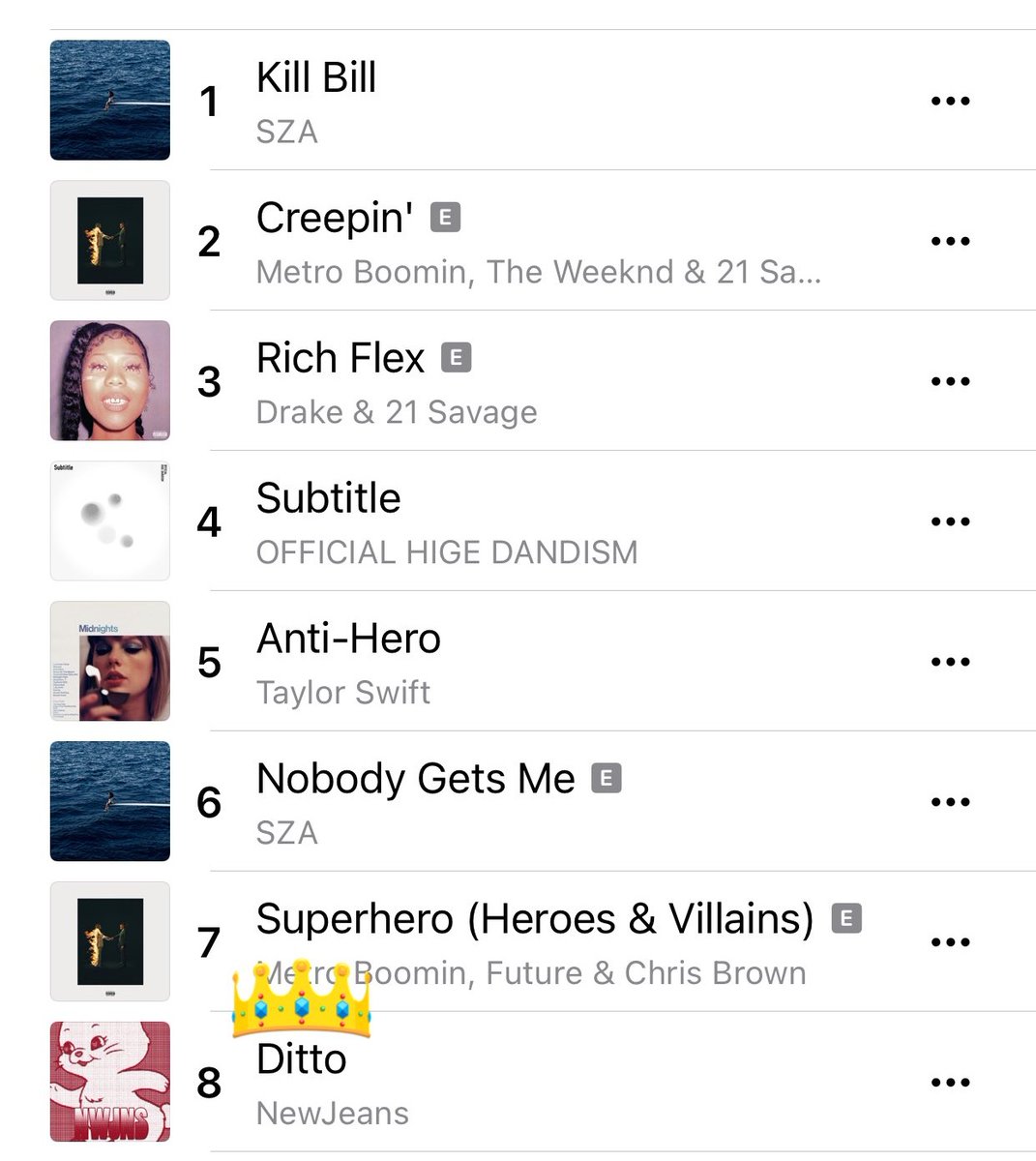This image is a screenshot from the Apple Music app showcasing a playlist with various songs. The detailed view includes the following:

1. **Kill Bill** by SZA - Showing her album cover on the left, with three dots next to it for more options.
2. **Creepin'** by Metro Boomin, The Weeknd, and 21 Savage - The album cover is displayed on the left with three dots for options.
3. **Rich Flex** by Drake and 21 Savage - Album cover on the left with option dots.
4. **Subtitle** by Official HIGE DANDism - Album cover on the left.
5. **Anti-Hero** by Taylor Swift - Featuring her album cover on the left.
6. **Nobody Gets Me** by SZA - The same album cover as "Kill Bill" on the left.
7. **Superhero (Heroes & Villains)** by Metro Boomin, Future, and Chris Brown - Album cover on the left.
8. **Ditto** by NewJeans - Album cover on the left, marked with a crown over the word "Ditto," suggesting it might be the user's favorite.

Each song entry features three dots on the right side, allowing users to choose various actions or settings for the tracks.